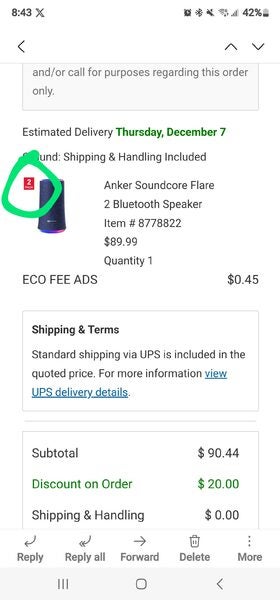A mobile device screen capture displaying a notification with a white background. In the upper left corner, the time reads 8:43. Directly below the time is a rectangular text frame with grey text stating, "and forward slash or call for purposes regarding this order only." Beneath this, in black and green text, it reads, "Estimated delivery Thursday, December 7. Shipping and handling included." On the lower left side of the screen, there is an image of a black Bluetooth speaker, highlighted within a green circle. To the right of the product description, the price is listed as 40 followed by "45 cents."